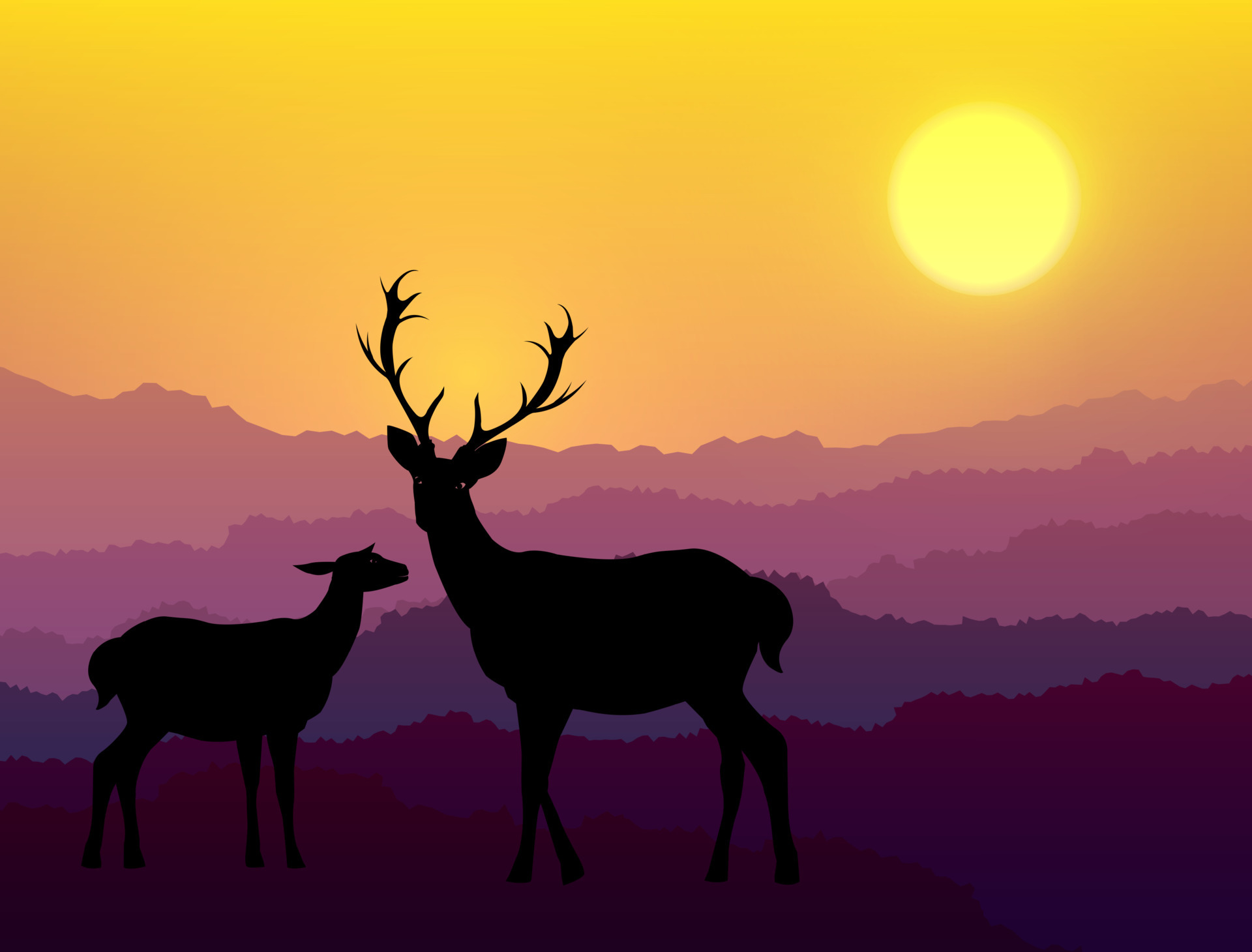The image is a computer-generated or cartoonish painting featuring two deer, depicted with smooth, computer-generated aesthetics. One is a larger deer with very long antlers, while the smaller one, likely a fawn or baby deer, is positioned next to the larger deer. The scene is set during sunset, with an orange sky and a yellow sun near the horizon, casting silhouettes of the deer in black. The background is kept simple with undefined ridges that could represent mountains or vegetation, colored in purples and pinks. The image has a minimalistic feel, focusing on the striking contrast of the silhouetted deer against the vibrant sunset.